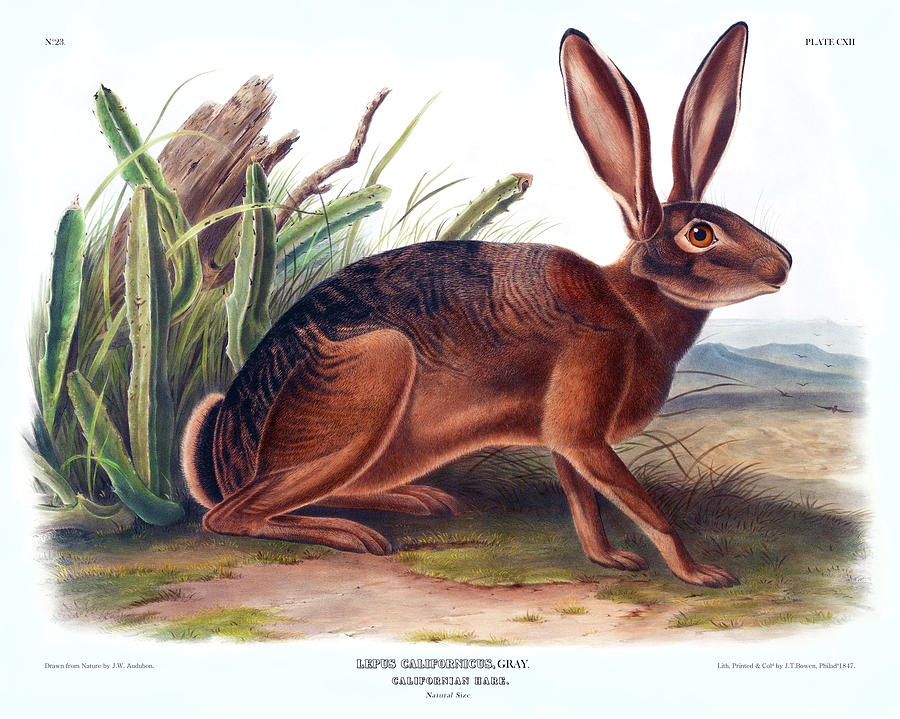In this detailed drawing, we see an exceptionally slender and elongated rabbit, facing right and presented in a side profile. The rabbit's fur is predominantly brown with black speckles along its sleek back. It has large, expressive brown eyes with a hint of orange, and similarly large ears that add to its distinctive appearance. The setting suggests a southwestern wilderness, characterized by a variety of natural elements: a patchy mix of grass and dirt underfoot, a cactus plant, and the remnants of an old wooden log. In the background, distant mountains and birds accentuate the desert-like atmosphere. Notably, the rabbit is identified in the inscription below the drawing as "Lepus californicus," or the rare Californian rabbit. The colors in the drawing are earthy and natural—browns for the rabbit, greens for the plants, and shades of brown and black for the surrounding elements, perfectly capturing the essence of this unique and graceful creature in its habitat.